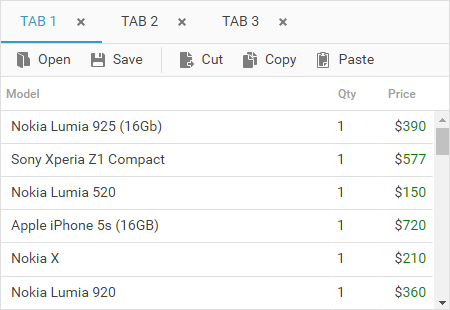Screenshot displaying three browser tabs with the first tab open. At the top of the interface, standard editing options are visible: open, save, cut, copy, and paste. The screen appears to be a tool for viewing or storing options.

The main content on the screen is a comparison chart of six cell phone models, each listed with its price and quantity. Detailed information includes:

1. Nokia Lumia 925 with 16GB storage - Quantity: 1, Price: $390.
2. Sony Xperia Z1 Compact - Quantity: 1, Price: $577.
3. Nokia Lumia 520 - Quantity: 1, Price: $150.
4. Apple iPhone 5S with 16GB storage - Quantity: 1, Price: $720.
5. Nokia X - Quantity: 1, Price: $210.
6. Nokia Lumia 920 - Quantity: 1, Price: $360.

The context suggests this is an inventory screen where someone is documenting or comparing prices and quantities of the listed cell phone models.